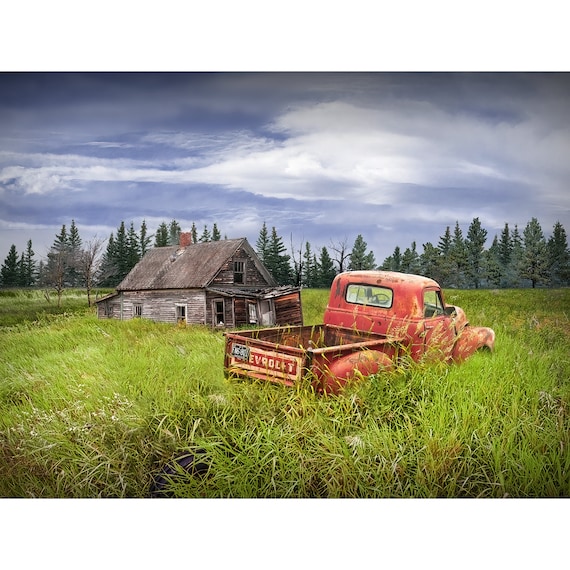The image depicts a desolate, rural landscape dominated by a dilapidated, weathered wooden house and an abandoned red Chevrolet pickup truck, surrounded by tall, unkempt grass. The worn, gray boards of the dilapidated house, which has a caving front room and a jutting chimney, suggest years of neglect. In the background, numerous stately pine trees provide a stark contrast to the rundown structures in the foreground. The sky above is a mix of clear blue and wispy cirrus clouds, adding to the serene, albeit abandoned, atmosphere. The scene feels cold and misty, enhancing the sense of abandonment and decay.